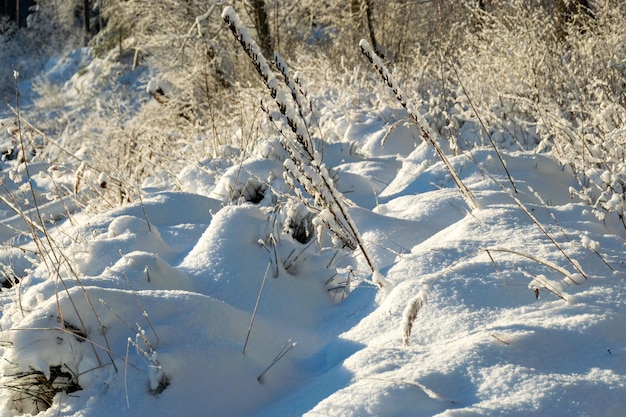The photograph, a detailed color image taken during winter, captures an outdoor scene blanketed with snow. The ground is uneven and lumpy with various mounds of snow, some of which form substantial snowbanks or drifts. Sticking up through the snow are numerous stalks of straw-colored wheat or a similar grain, giving it a yellowish-gold hue amidst the predominant bluish-white snow. The sun is shining brightly, casting distinct shadows across the snow, adding depth to the scene. The background is filled with thicker vegetation, suggesting the photo was taken in a wooded area or forest. The snow appears untouched by human or animal tracks, reinforcing the serene, undisturbed nature of the setting. Where the snow has settled on branches and sticks, there are intricate details of accumulated snowfall adding texture to the image.